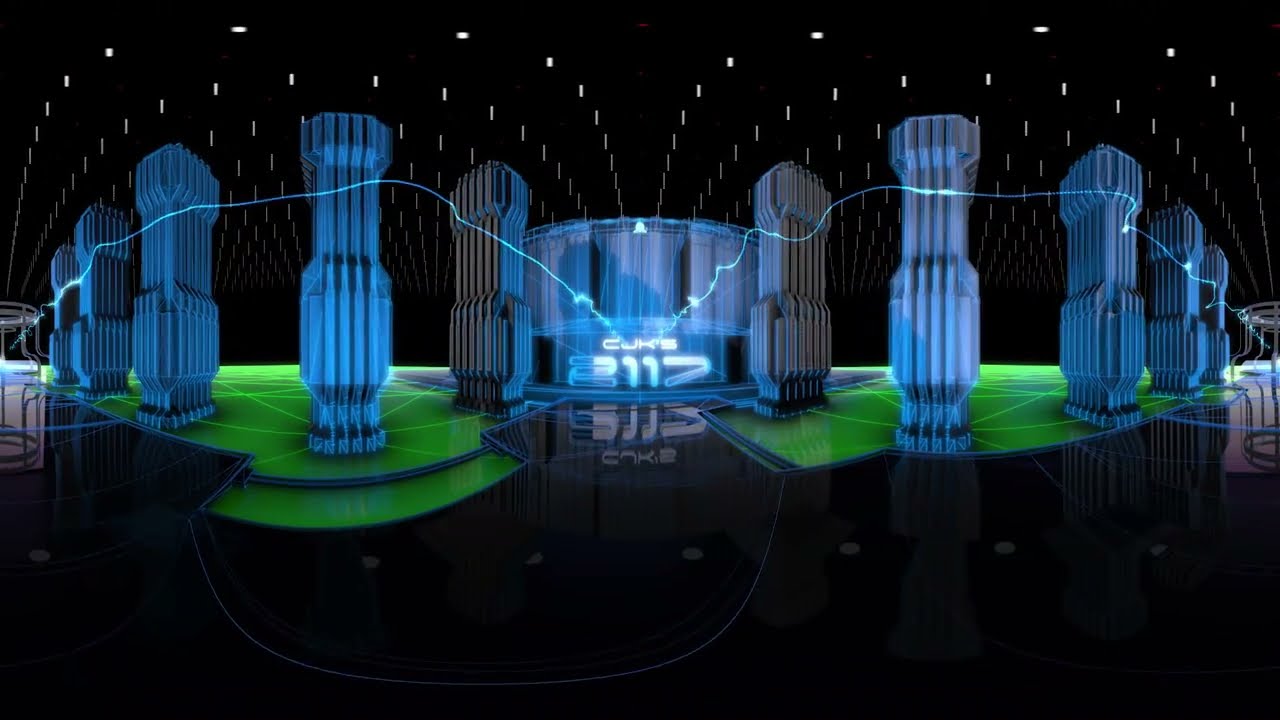The image depicts a black background with a primarily black floor, partially accented with green areas that have lines running through them. Dominating the scene are multiple tall, blue digital columns arranged symmetrically, with four columns on each side. At the center of the image, two blue columns flank a spherical neon object that bears the glowing inscription "CJKS2117." This central sphere is mirrored in the black floor below it. Radiating from the sphere is an electrical shock-like blue line. The columns and sphere are surrounded by several white dots that seem to align with the columns' arrangement. Above the scene, the sky is black, dotted with numerous rectangular lights. The overall ambiance suggests an entrance to a futuristic or digital temple-like structure, possibly within a video game environment.